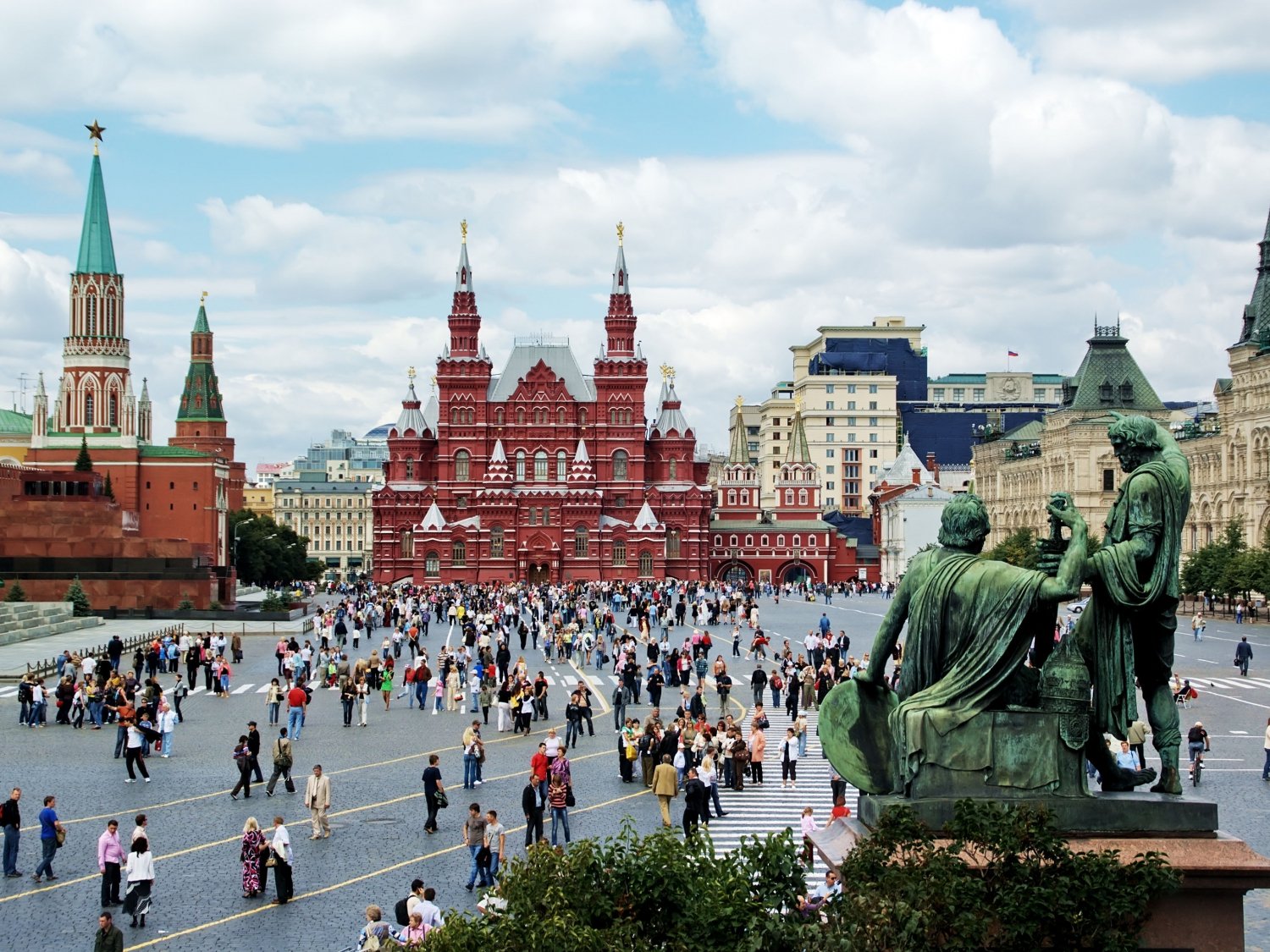This striking cityscape photograph captures a bustling foreign metropolis from an elevated vantage point. The scene is vibrant and full of life, featuring an array of tall, colorful buildings in shades of white, blue, brown, beige, and pink. A standout structure in the center is a burgundy building with white peaks, topped by a blue or green spire adorned with a star. The sky above is bright blue and dotted with large, fluffy white clouds, adding a dramatic backdrop to the urban setting.

In the foreground, a green statue of two men draws attention—they face away from the viewer, one standing and the other sitting. The statue is positioned on a wooden platform next to lush green trees and leafy bushes, enhancing the contrast between nature and the bustling urban environment. The streets below are teeming with people dressed in colorful attire, suggesting a popular tourist attraction or city center. The atmosphere is lively and dynamic, with numerous individuals walking, standing, and engaging in conversations amidst the architectural splendor of this diverse city.